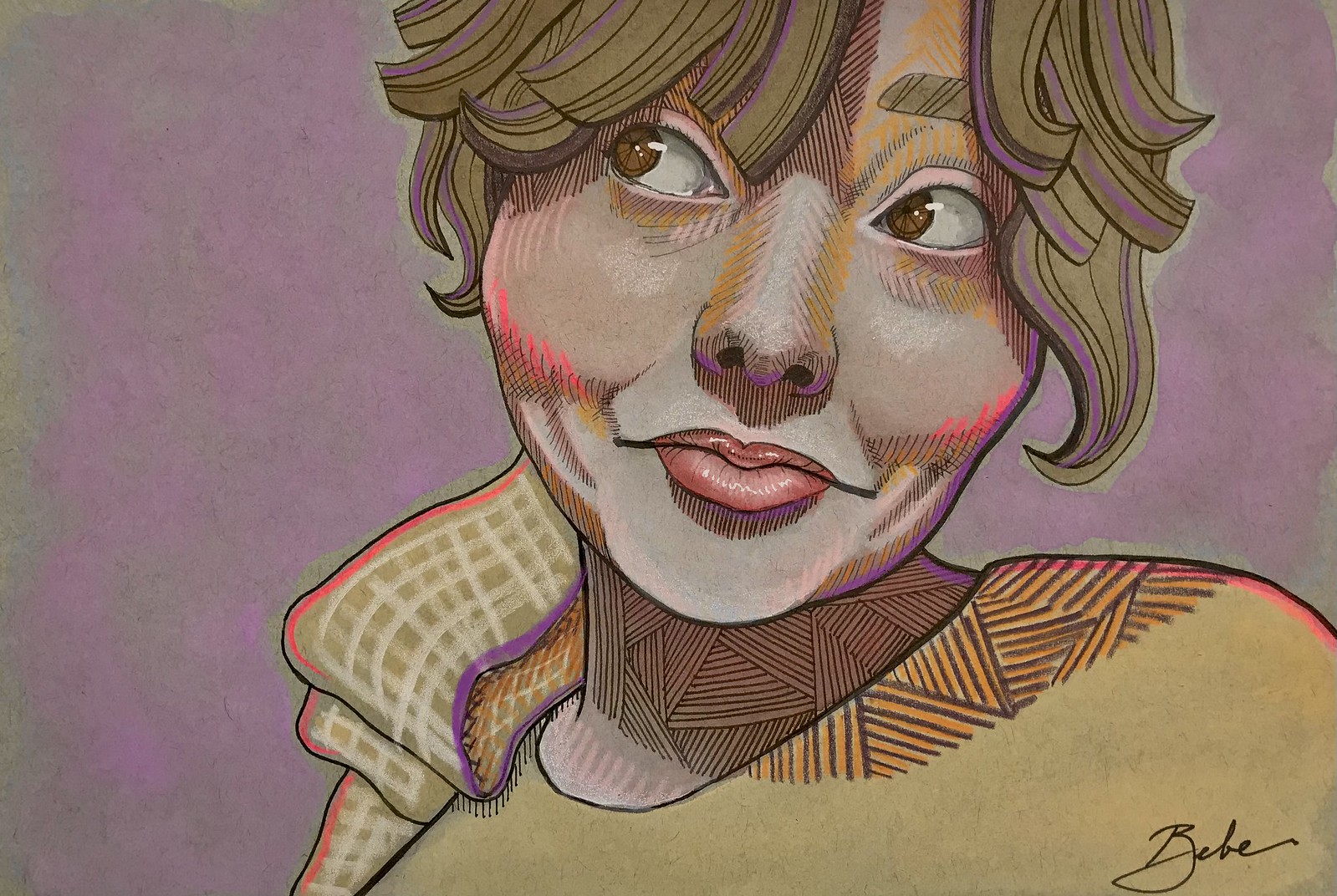This detailed and realistic digital illustration, signed by the artist "B.E.B.E" in cursive in the lower corner, portrays a young woman against a background of purplish gray hues with touches of greens, adding depth and shading through cross-hatching techniques. The woman, depicted from just above her eyebrows to just below her shoulders, appears to be tilting slightly to her right. Her expressive face is turned to the left, showing her brown eyes looking pointedly to the right, suggesting an amused yet doubtful interaction. Her eyebrows are raised and her lips, colored red with white highlights, form a slight, downturned smile.

She has brown hair, styled with a fringe of bangs framing her face and a loose strand falling over her cheekbones, while the rest is pulled back, giving her hair a textured, flat pasta-like appearance. She wears a round-neck top in shades of yellow to light brown, featuring a pattern of alternating triangles at the neckline. Adding a charming detail, a light brown bow adorned with a grid of light yellow squares and edged in a pink to orange hue hangs from the nape of her neck. The realistic rendering accentuates her high cheekbones and subtly highlights her skin tones on her face and neck, creating a lifelike effect. The overall composition balances intricate details and expressive elements, making the portrait captivating and personable.